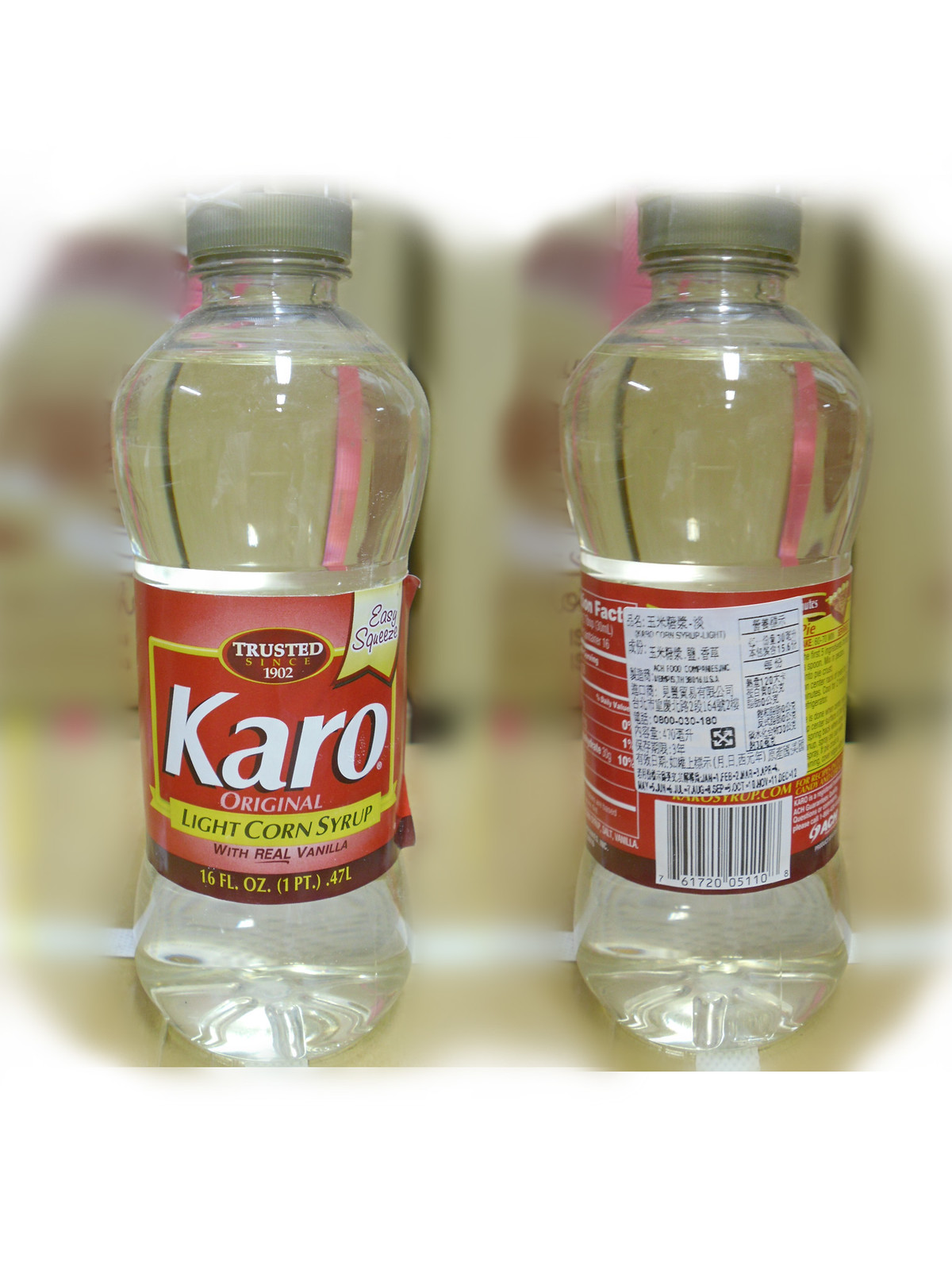This is a color photograph of two bottles of Karo Original Light Corn Syrup, both 16 fluid ounces (0.47 liters) with gray caps, and filled with a clear liquid. The bottle on the left prominently displays the front label, which is a combination of red, white, and yellow, and reads "Trusted since 1902, Easy Squeeze, Karo, Original Light Corn Syrup with Real Vanilla." The bottle on the right shows the back label, featuring nutrition facts and a barcode, partially obscured by a white sticker with an Asian language translation. The background of the photograph is blurred, with the image fading out at the top and the bottom corners.